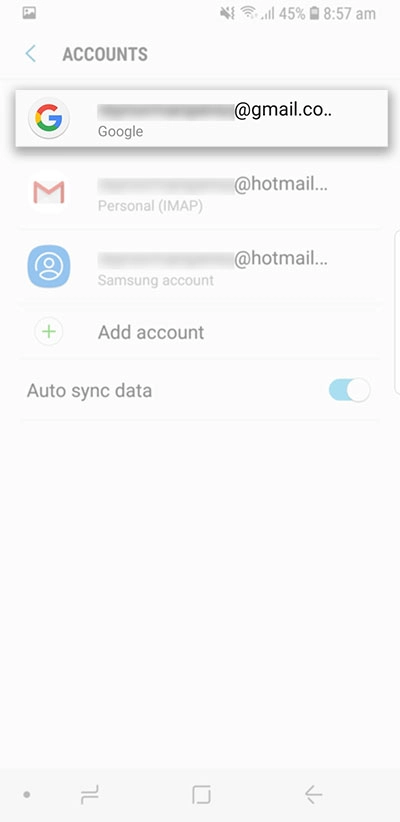The image displays an account management page on a mobile device. The screen's bottom section features a slightly darker gray border housing four distinct icons. From left to right, these include a gray dot, a pair of overlapping L-shaped icons (one pointing up to the right, the other pointing down to the left), an empty square, and a back arrow pointing to the left.

At the top, the status bar shows several indicators: an images icon on the upper left, a no sound notification icon, Wi-Fi, data indicators, and a battery life indicator showing 45% in gray, all located on the upper right. The time is displayed at 8:57 AM.

Directly below the status bar, a blue left-pointing arrow is labeled "accounts." The page lists three accounts with their respective details:

1. A Google account, represented by a Google "G" profile image, with "at Gmail.co" and "Google" written underneath in gray.
2. An email account marked by a mail icon, labeled "at Hotmail," followed by "personal IMAP" grayed out.
3. Another "at Hotmail" account, denoted as a Samsung account, also grayed out.

At the bottom of the account list, there's a green plus button labeled "add account" and an auto-sync data option, which is checked on.